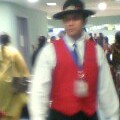The image is a small, blurry photograph capturing a scene with multiple people in a wide, open area with white walls and bright white ceiling lights. The focal point of the image is a man of apparent Mexican descent, dressed in an elaborate costume. He is wearing a white collared long-sleeved shirt, a vibrant red vest, a blue tie, and a black wide-brimmed hat with a distinctive bolo-style center. Around his neck, a lanyard hangs, bearing an out-of-focus white badge.

To his left stands a person with brown hair tied into a ponytail, wearing a large white coat or possibly a trench coat. In the background, a woman in a yellow dress or coat with long hair can be seen, and she appears to be holding something silver. Additionally, another person can be perceived wearing what looks like a cheetah print dress. The area teems with numerous people, suggesting the setting might be a busy mall or shopping center. On the left side of the image, there is a door that appears to be gray or slightly light purple, though the low resolution makes it difficult to pinpoint exact details.